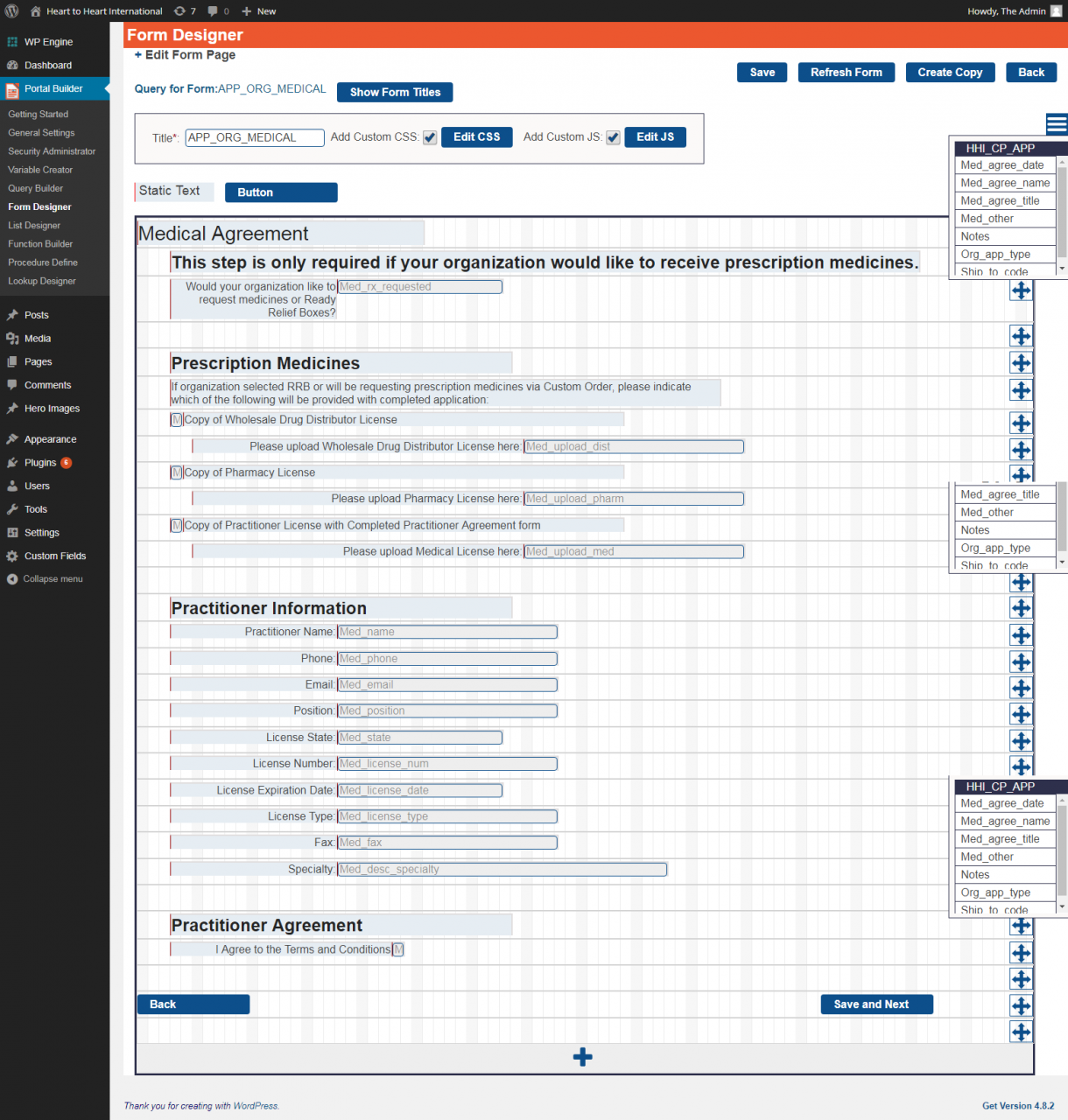The image depicts a section of a web application, likely designed for organizational use. The interface is dense with text and includes various functional elements. On the left sidebar, which features a black background, multiple menu options are visible. These include "Heart2Heart International" at the top, followed by categories such as "WP Engine Dashboard," "Portal Builder" (highlighted in blue), "Form Designer" (currently the active section), "Getting Started," "General Settings," "Security," "Variable Creator," "Query Builder," and more. Additional options like "Posts," "Media," "Pages," "Comments," "Hero Images," "Appearance," "Plugins," "Users," "Tools," "Settings," "Custom Fields," and "Custom Collapse Menu" are also listed.

The main content area is centered on the "Form Designer" section, which is enclosed within an orange box. This section provides numerous editing options with buttons at the top labeled "Show Form Titles," "Save," "Refresh Forms," "Create Copy," and "Back." The form in view appears to be a medical agreement form, specifically addressing the provision of prescription medications. One part of the form states, "This step is only required if your organization would like to receive prescription medications." Below this, there's a checkbox question asking whether the organization would like to receive such medications, followed by sections labeled "Prescription Medications" and explanations about requesting medications via a custom order.

Further details include fields for indicating funding sources and uploading various licenses (wholesale drug distributor license, pharmacy license, practitioner license). The form also requires practitioner information such as name, address, licensing details, email, and position, along with a "Practitioner Agreement" section where the practitioner must agree to terms and conditions. At the bottom, there are navigation buttons with "Back" on the left and "Save and Next" on the right. The form is intricate, with numerous checkboxes and text fields, indicating a complex and detailed data entry process.